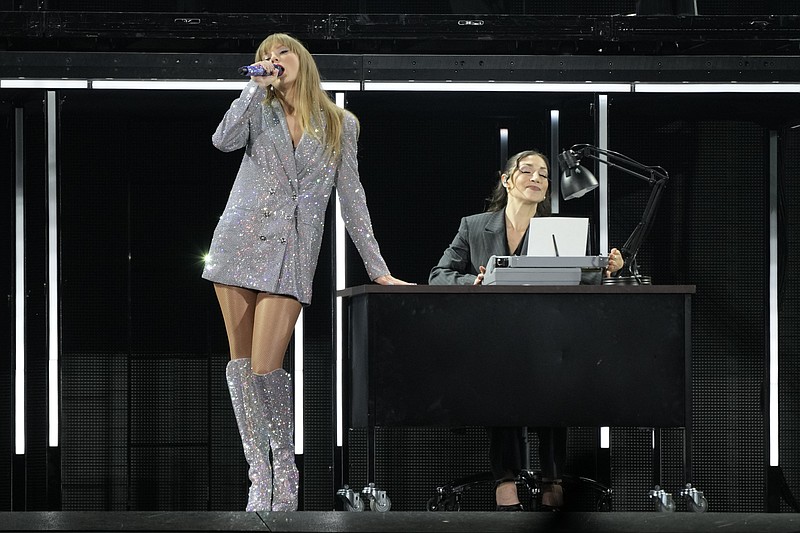In the image, Taylor Swift is depicted mid-performance, standing to the left of a stylish office desk on a multi-level stage. Her long, flowing blonde hair with bangs cascades down to her shoulders, and she captivates the audience with her voice, singing into a microphone held in her left hand. Taylor's ensemble is striking—a bejeweled, bedazzled, sparkly silver jacket paired with knee-high matching boots, both adding a glamorous touch to her presence. The desk next to her is black with a wood finish top and sits on four caster wheels. A woman dressed in a black business suit is seated behind the desk, seemingly engrossed in typing on a typewriter-like device. This desk setup includes a small swing arm lamp, enhancing the office-like appearance. The woman serves as a prop, portraying an office worker, adding an intriguing element to Taylor Swift's performance.